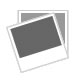The image showcases a collection of five antique, rusted metal handles, each with its own unique characteristics. Starting from the top, the first pair consists of shorter handles with flat ends, each featuring two holes for mounting, indicative of a uniform design likely from the same manufacturer. The second pair, slightly longer, displays a distinct design with scalloped ends, adorned with three rounded points, and three mounting holes on each end, also suggesting they were produced together. The final, solitary handle at the bottom, is the longest of the collection and resembles a standard cabinet handle with flat ends, though it deviates by having only one mounting hole on each end. All the handles are heavily rusted, with a patina indicating extensive use and considerable age, adding to their vintage charm. The varied designs and wear patterns suggest they were once part of different pieces, possibly from doors, drawers, or suitcases, giving an air of nostalgic craftsmanship to the collection.